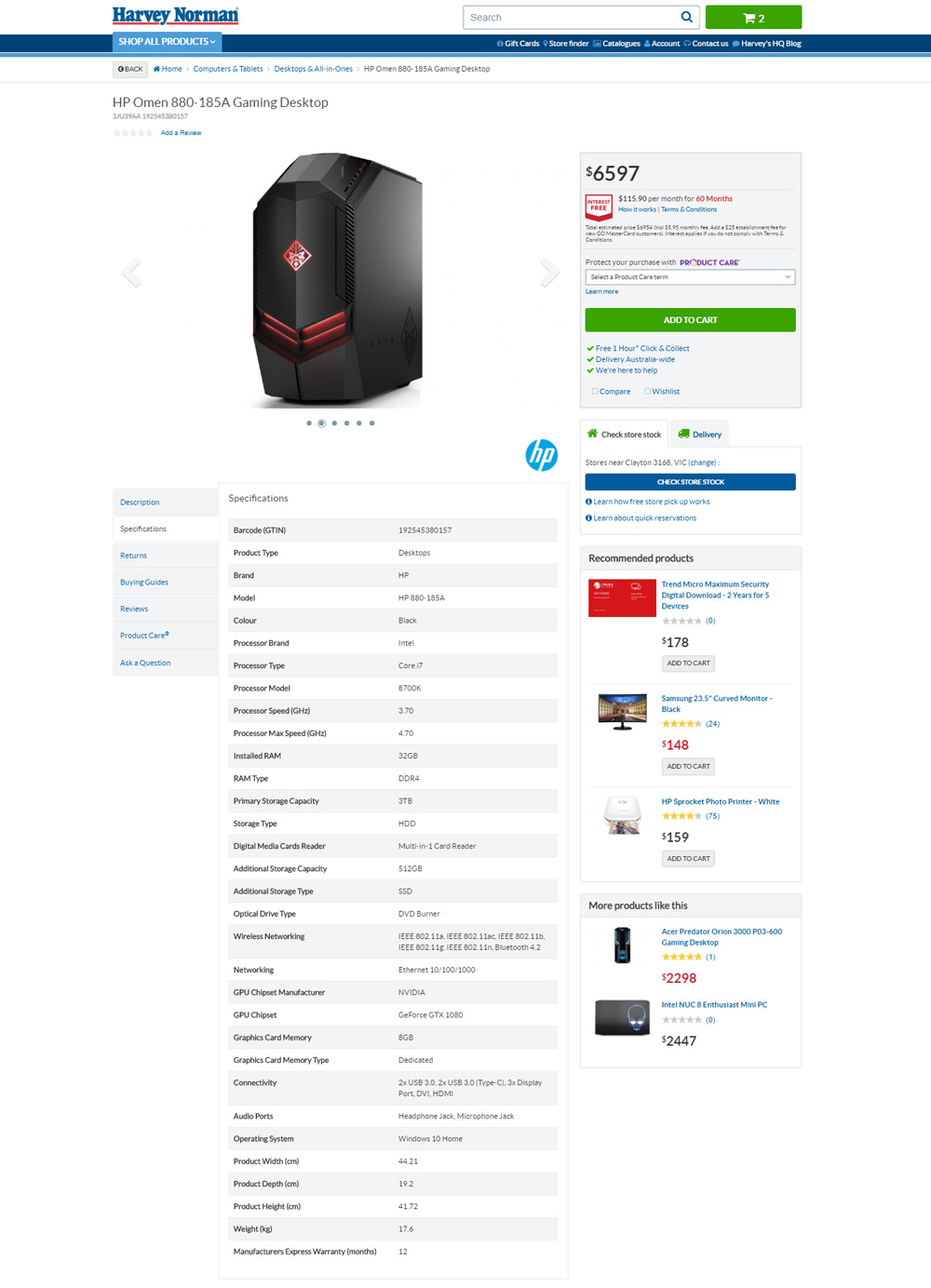A detailed screenshot from the Harvey Norman website, displayed on a desktop monitor. Positioned at the top left of the webpage is the recognizable Harvey Norman logo, while directly to its right is a functional search bar. The webpage prominently features an HP Omen 880-185a gaming desktop, tagged at a premium price of $6,597. Centered on the page is an exhaustive list of the gaming desktop's specifications, presented in a structured format under the active "Specifications" tab. To the left of the product details is a narrow menu showcasing additional navigation options, though the text is too small to discern clearly. On the far right side of the screen, there's a column dedicated to recommended and similar products, all of which are more affordable alternatives to the featured HP Omen 880-185a. The webpage captures the entire layout of the product listing, providing a comprehensive view of the detailed specifications and additional consumer suggestions.